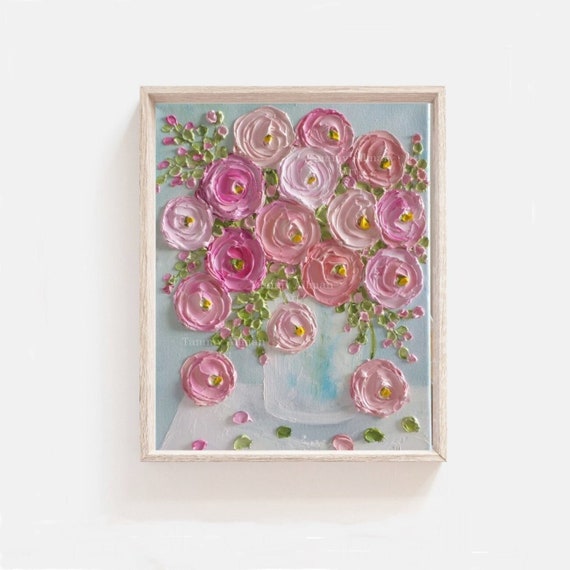The image depicts a photograph of a textured painting centered on a white wall. The painting is framed by a light, thin wooden frame and showcases a vase with an arrangement of pink flowers resting on a white table. The flowers, rendered with thick, swirling strokes of paint, present a 3D texture, featuring rosettes in various shades of pink with subtle yellow centers, accompanied by green leaves. Some petals and leaves appear to be falling, adding to the lifelike quality. The painting's background is a light blue color, enhancing the vibrant pinks and greens. The textured and intentional brushwork suggests a special painting technique, offering a visually striking and detailed floral composition.